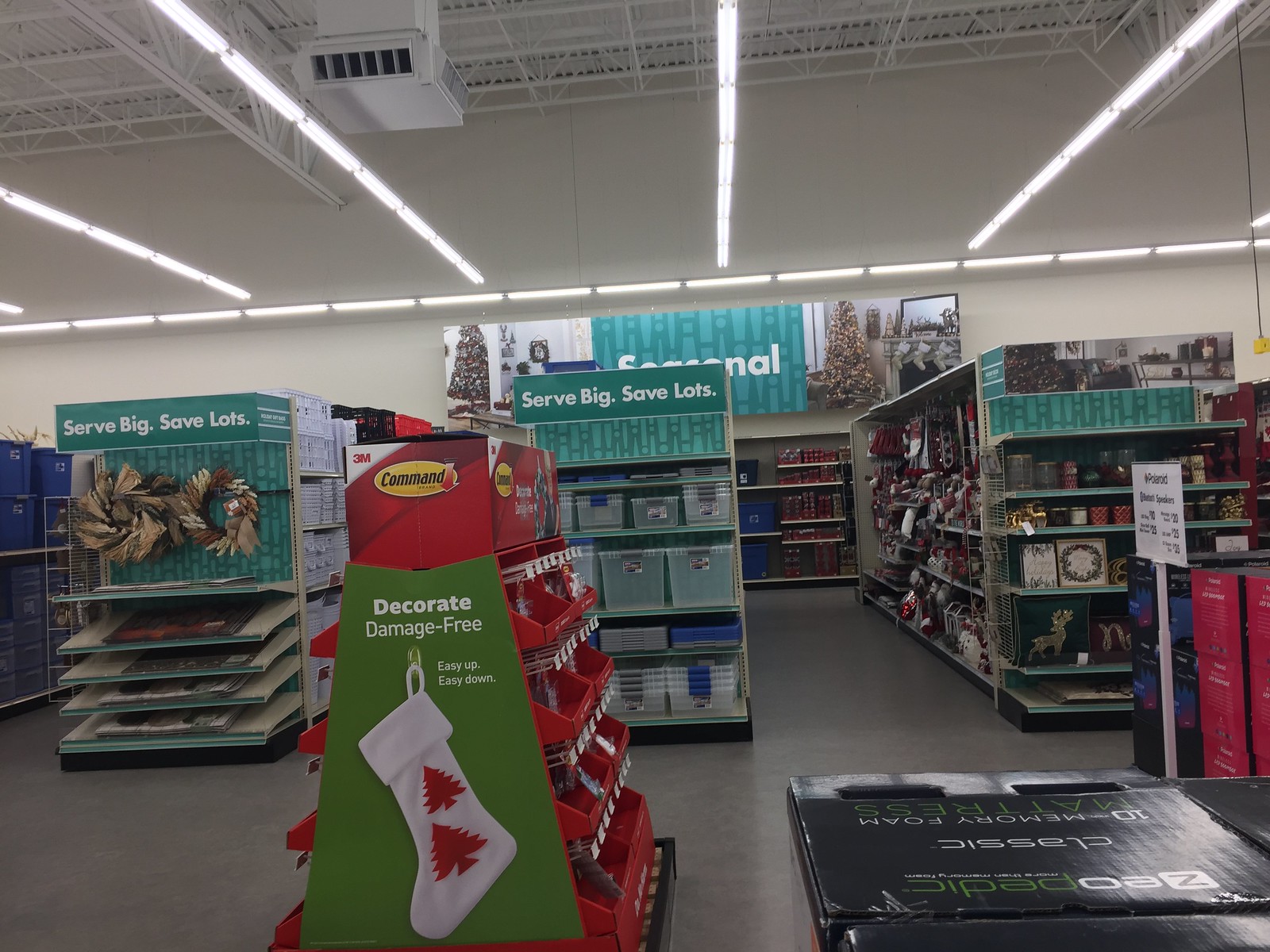The photograph, likely taken inside a department store, captures the ambiance of a craft or decorative section during Christmastime. The store exhibits high ceilings adorned with commercial fluorescent lighting, providing a well-illuminated space. Visible in the photo are multiple racks organized with various items: one rack displays festive wreaths, another holds storage bins, and a third is dedicated to assorted Christmas decorations. Signage indicating the seasonal theme, including images of Christmas trees, adds to the festive atmosphere. Prominent banners at the top of two racks read "Serve Big, Save Lots," suggesting the store may be a Big Lots location. Additionally, a standalone red rack featuring Command products, such as hooks and hanging devices, is seen in the aisle. The photo is taken from the aisle's end, offering a comprehensive view down the row of meticulously-arranged holiday merchandise.